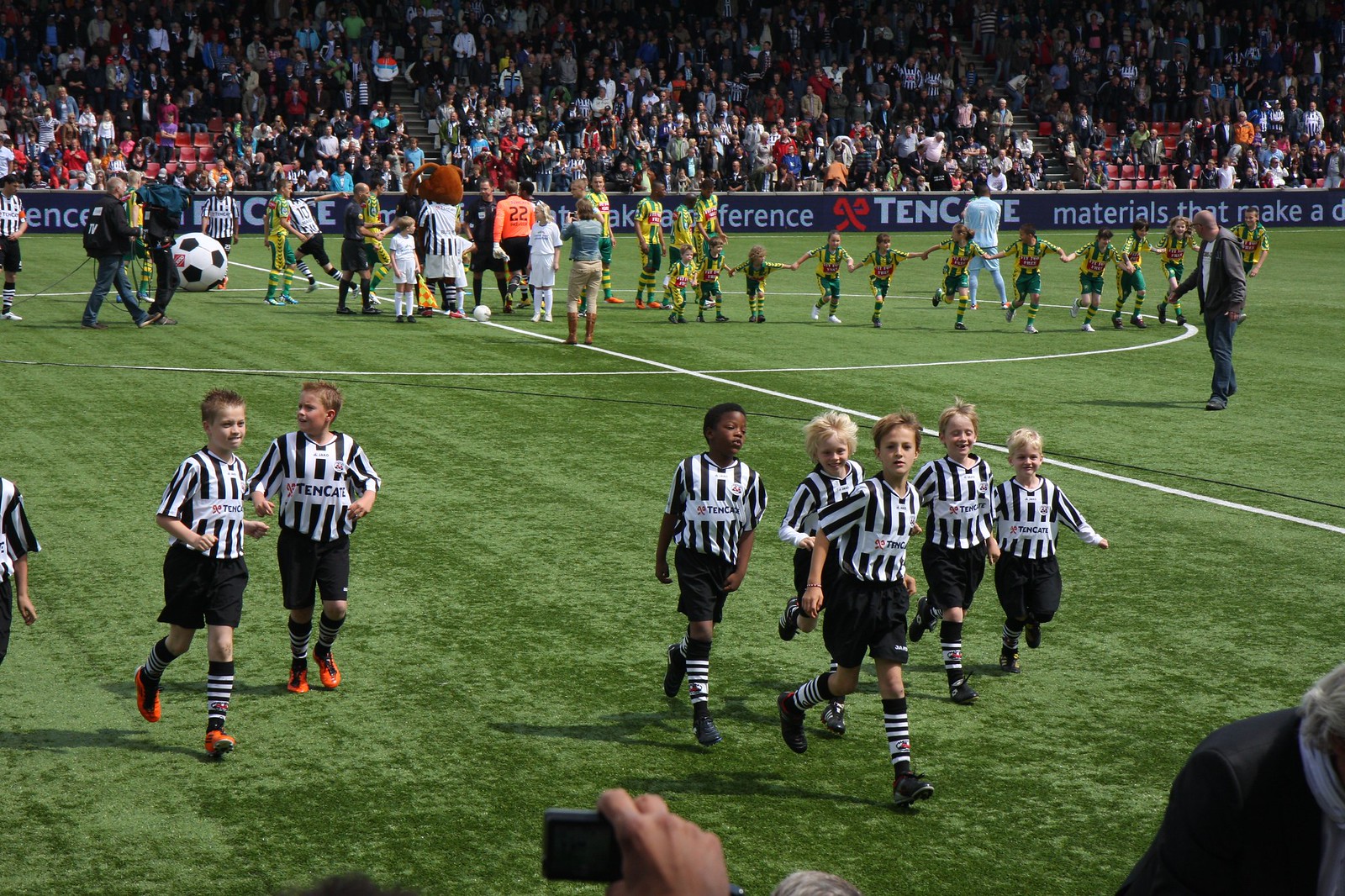The image depicts a vibrant and lively scene on a green grassy soccer field marked with white lines. In the foreground, seven or eight young boys, estimated to be around seven or eight years old, are energetically running toward the front. They are dressed in coordinated black and white vertical striped shirts, black shorts, and matching black and white striped socks. Their expressions of joy suggest they are having fun, possibly running off the field. 

In the background, there is another group of children wearing yellow and green uniforms, holding hands and appearing to run towards the same sideline. Between these groups of children, some adults are visible, along with a mascot dressed in a colorful outfit, adding to the festive atmosphere. A giant soccer ball can be seen in the air above the scene.

Further back, a large audience is seated in the stands, though their details are not in focus. The overall setting resembles a stadium during a daytime event, filled with excitement and activity.